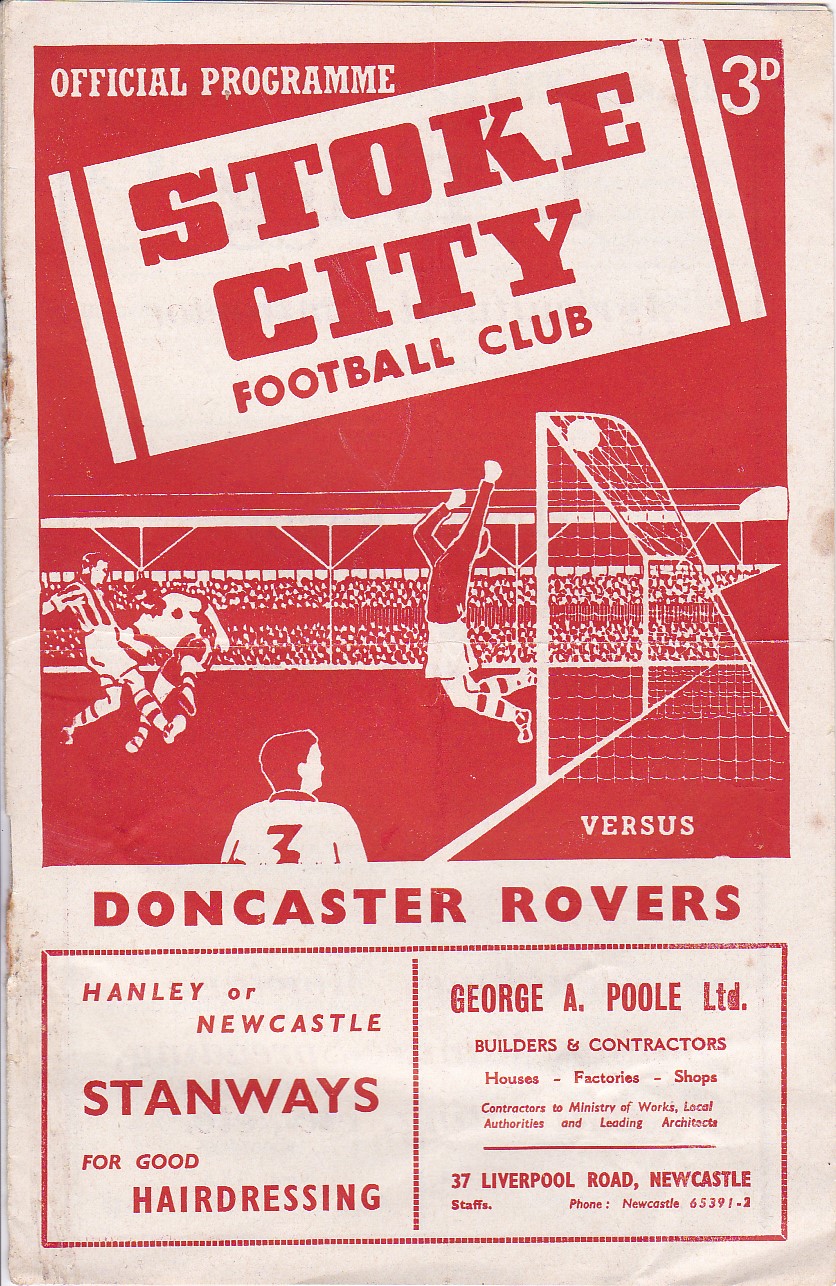This poster is an official program for a Stoke City Football Club match against Doncaster Rovers. The poster features a white border with a dominant red center. At the top, in white lettering, it reads "Official Programme" (with the British spelling). Additionally, near the right corner, there's a small "3d" indicating the price, and a white, ticket-like rectangle, slightly crooked, displaying the title "Stoke City Football Club."

The central image in the red square depicts a scene from a soccer match. A football player with his back turned, wearing a white jersey emblazoned with a red number "3", is captured in action. He is kicking a ball towards the goal. The goalie's posture indicates an attempt to block the incoming shot; the goalie is dressed in a red shirt and white shorts. The net in the goal is white, complementing the overall color scheme of red and white.

Below the image, text reads "vs Doncaster Rovers," indicating the teams competing. The bottom section of the poster includes advertisements: one for "Hanley or Newcastle Stanways for Good Hairdressing," and another for "George A. Poole LTD, Builders and Contractors" complete with an address at "37 Liverpool Road, Newcastle" and a phone number "Newcastle 653912." The overall design suggests a historical, promotional material for a football event, emphasizing the timeless red and white club colors.